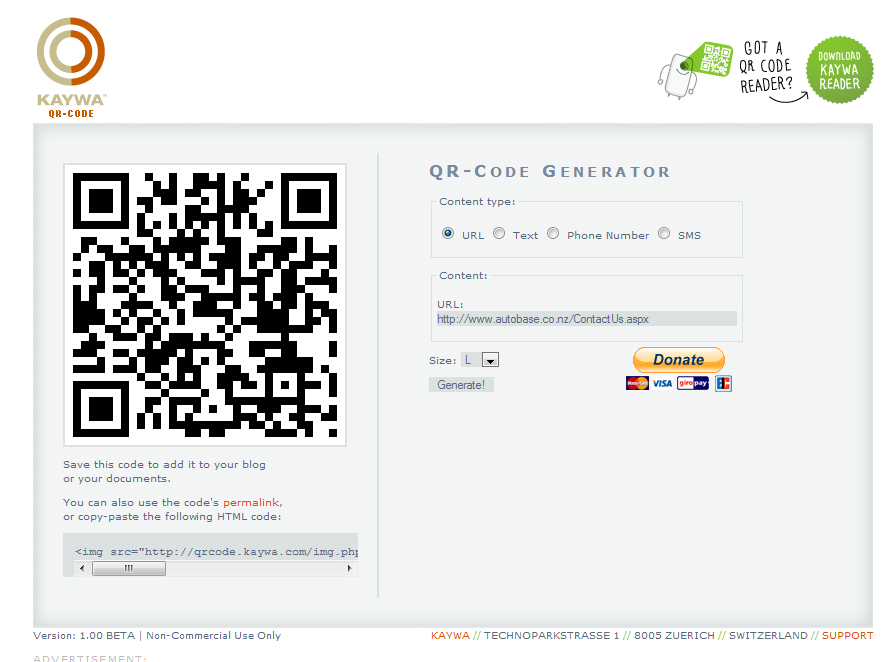The image depicts the Keiwa QR Code generator interface. At the center, two concentric rings are partially colored with beige on the left and orange on the right. In the top right corner, a small phone-like character emits a QR code, with the text "Got a QR code reader?" in black pointing to a green circle labeled "Download Keiwa reader."

Below this, on the left side, there is a gray box containing a QR code alongside the instruction, "Save this code to add it to your blog or your documents. You can also use the code's permalink." The word "Permalink" is highlighted in orange, followed by "Copy-paste the following HTML code," with an editable HTML code box beneath it.

On the right side, the interface includes a section titled "QR Code Generator." Here, users can select the content type from options such as URL, Text, Phone Number, or SMS, with the URL option highlighted. Beneath this, the content field displays "URL: autobase.co.nz/contactus.aspx." Users can then choose the size "L" and click "Generate" to create their code.

Additionally, there is an orange "Donate" button, supported by logos for MasterCard, Visa, Giropay, and BC located at the bottom, indicating accepted payment methods.